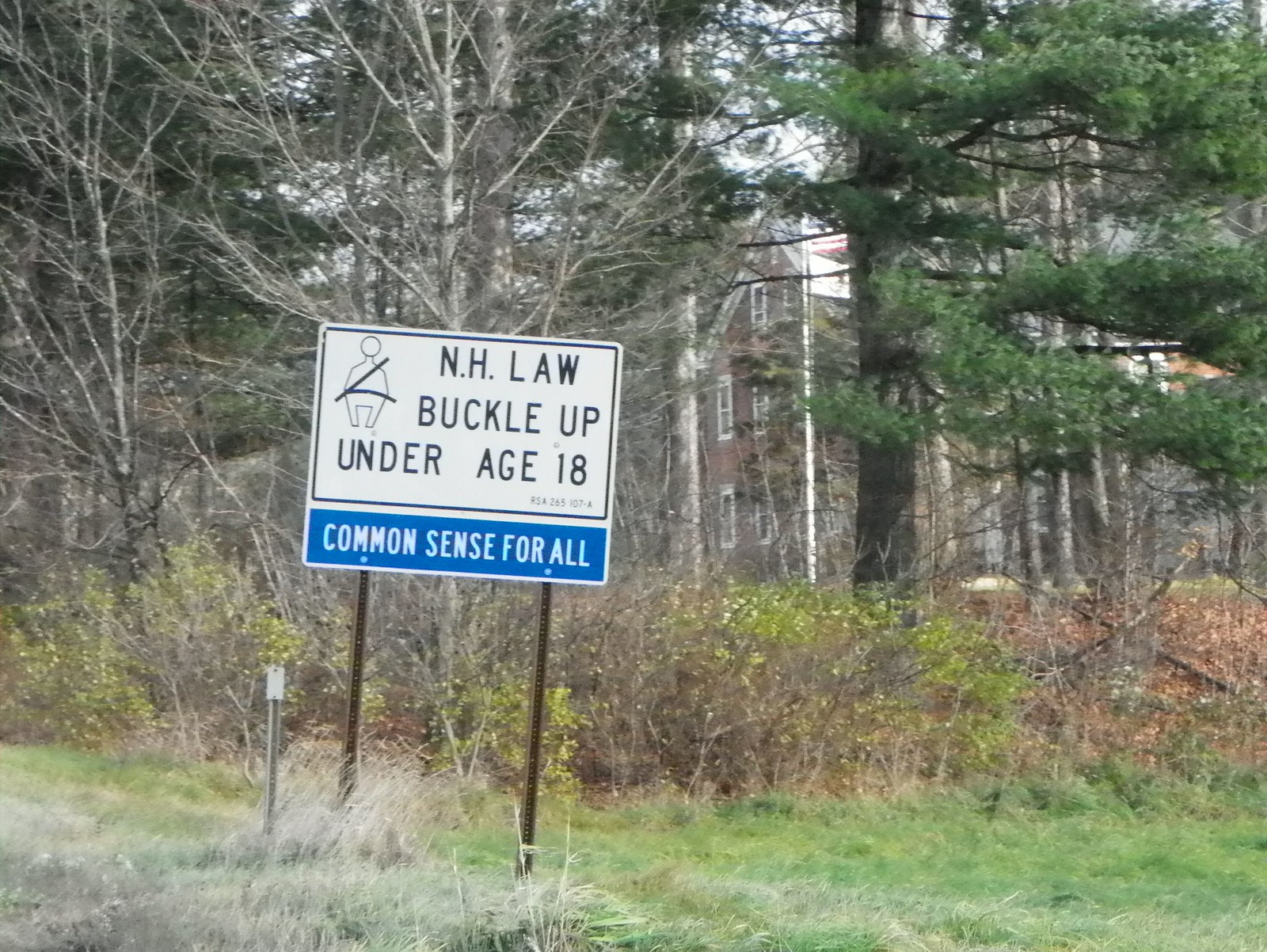This vibrant color photograph, captured during the day from a roadside, vividly showcases a grassy area dotted with bushes. Dominating the foreground is a notable roadside sign. The upper part of the sign is white with black lettering, stating, “NH Law Buckle Up Under Age 18,” accompanied by a simple illustration of a person wearing a seatbelt. Directly below, a blue sign with white lettering proclaims, “Common Sense for All.” The backdrop of the image features dense bushes and tall, majestic trees, through which glimpses of a large, historic building are visible. The partially visible structure, resembling an old farmhouse or a historical edifice, appears to be three stories high with a brown or brick facade and accented by white windows, adding depth and context to the scenery.